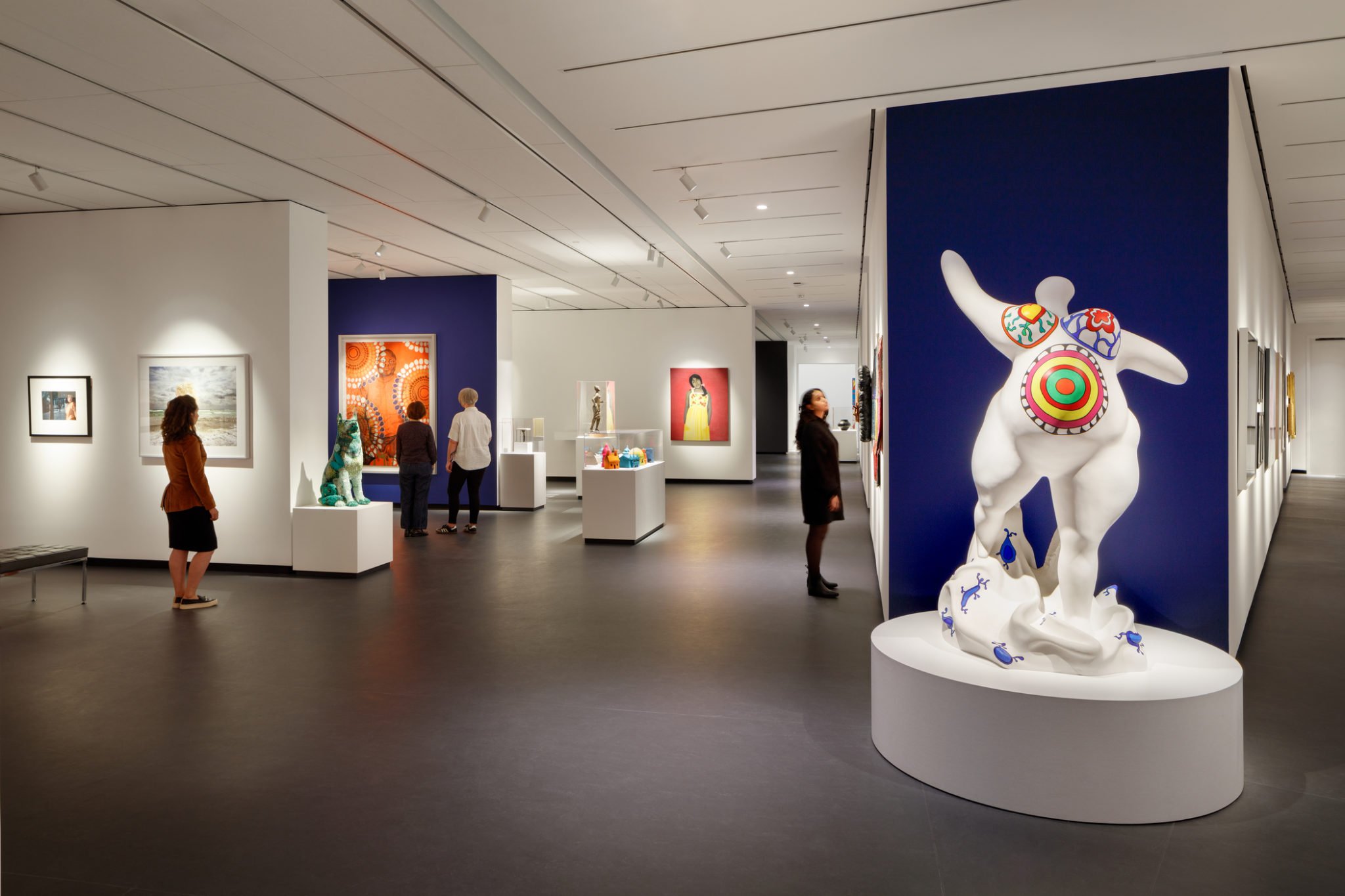The image captures an art gallery setting filled with various pieces and human interaction. In the foreground, a man and a woman are closely examining a blue-painted cubicle adorned with intricate artworks, one of which features circular patterns. The man is attired in a white shirt, blonde hair, and black pants, while the woman wears a brown sweater with black pants. They are engrossed in a sizable painting on the blue wall. 

In the middle, a glass-top display sits on the gray floor, containing vibrant blue and red elements. To the left, a white cubicle houses two distinct pieces illuminated by overhead lights: a face sculpture and a quirky figure of a dog topped with green foam. Standing by this cubicle is one of the gallery visitors, adorned in a brown blazer and black skirt, captivated by the art.

On the far right, under the white ceiling with attached lights, stands an imposing white statue of a person without a head. This figure, seemingly female, is elaborately detailed with colorful target-like markings in green, red, yellow, and blue across its torso, emphasizing the belly and breasts. Nearby, a woman in an all-black ensemble, including a coat and shoes, gazes thoughtfully upwards.

An additional figure, clothed in a black coat and black shoes, also takes in the surroundings. Lastly, the far wall displays a striking painting of a woman in a yellow dress set against a vivid red backdrop. Throughout the gallery, there are framed pictures and various other artworks, showcasing a rich mix of colors and styles, providing a bustling yet contemplative atmosphere indicative of an art exhibit.